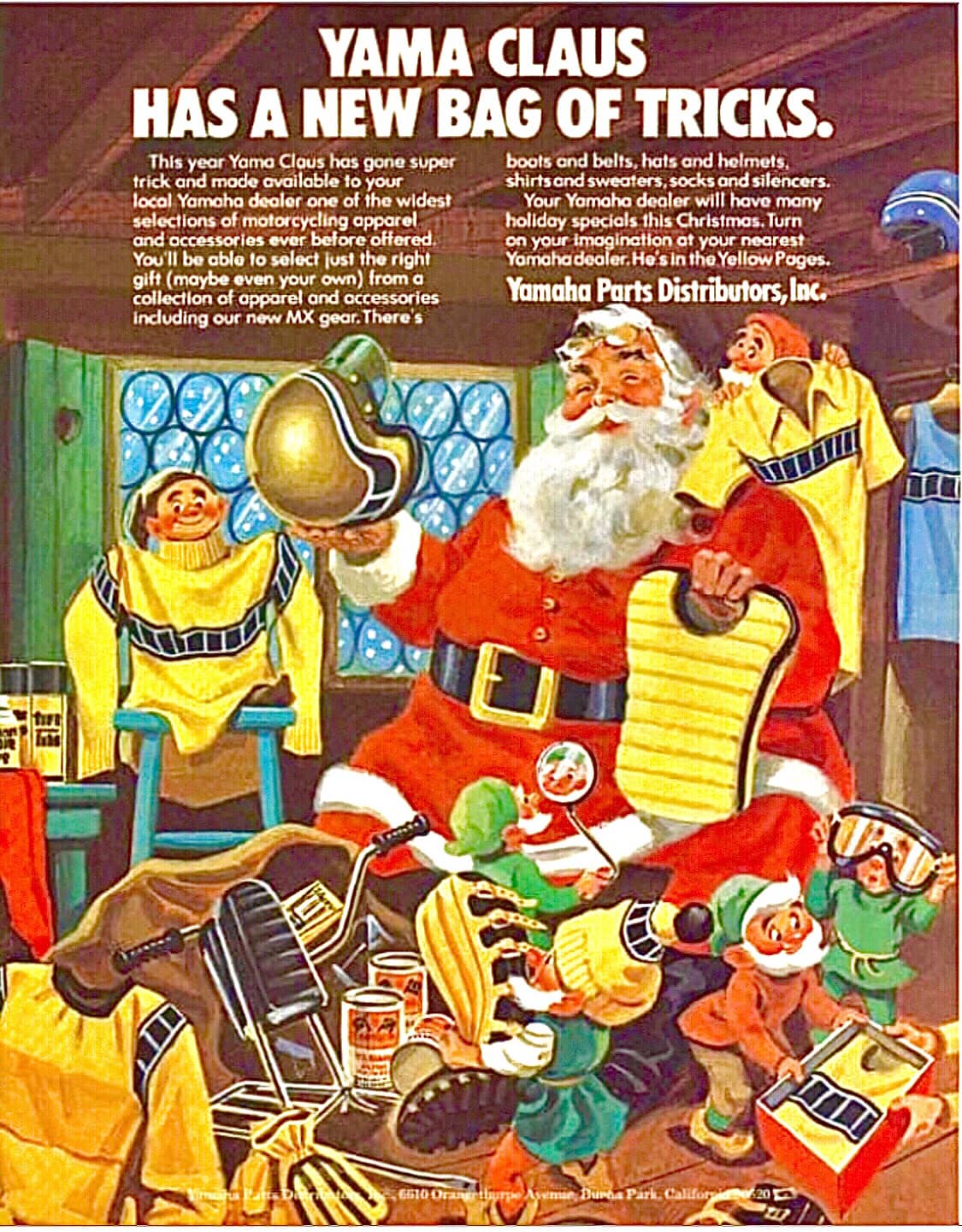This is a tall, rectangular image resembling a cartoon-style poster, primarily serving as an advertisement for Yamaha during Christmastime. The central focus is a colorful painting of Santa Claus, prominently positioned on the right side. Santa is a large figure, dressed in his traditional red outfit with white trim, a big black belt with a gold buckle, and a long white beard. Uniquely, he’s depicted with sunglasses perched atop his head.

Santa is seated, surrounded by a bustling scene of elves eagerly preparing gifts. One elf, standing on Santa’s left, is wearing an oversized yellow sweater with a blue stripe across it, comically too large for him. Another elf behind Santa holds up a yellow shirt featuring a white stripe across the front. In front of Santa, a group of elves is engaged in wrapping more yellow sweaters with blue stripes, while an array of objects including cans, gloves, eye goggles, and a gold helmet scatter the ground around them. At Santa's feet, there's also a sack with handlebars of a motorcycle peeking out, emphasizing the advertisement’s connection to Yamaha.

The top of the poster reads in bold white letters, "Yama Claus has a new bag of tricks." Below, the text elaborates, "This year Yama Claus has gone super trick and made available to your local Yamaha dealer one of the widest selections of motorcycling apparel and accessories ever before offered." The description promises a wide variety of gifts, mentioning items such as boats, belts, hats, helmets, shirts, sweaters, socks, and silencers, all available at Yamaha dealers, which the text notes can be found in the Yellow Pages. Another paragraph to the right further promotes Yamaha's extensive holiday specials, urging readers to turn on their imagination this Christmas at their nearest Yamaha dealer.